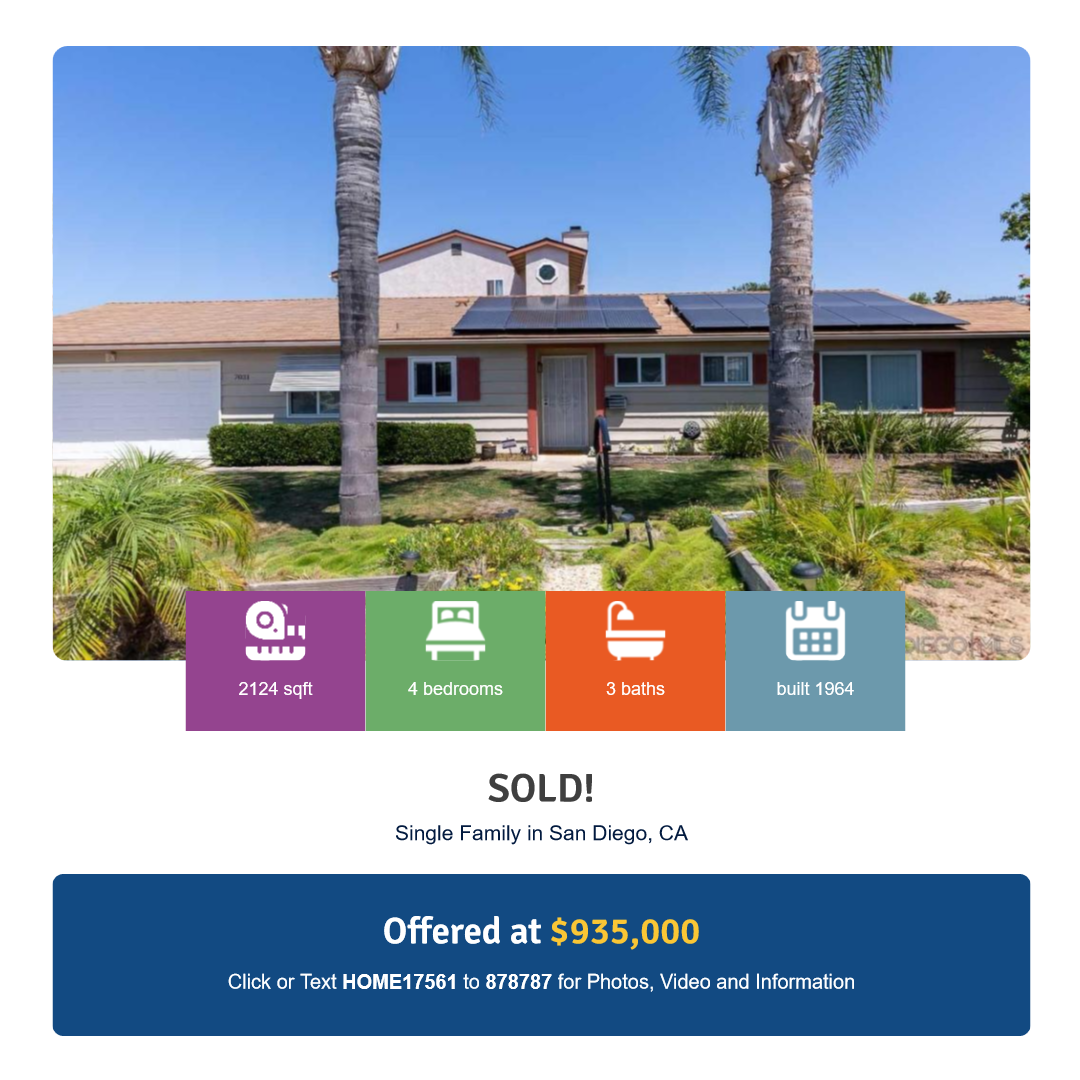A vivid image from a home sales website showcases a charming single-story house, highlighted by environmentally-friendly solar panels adorning its roof. Two towering palm trees add character to the front yard, which is also beautifully landscaped with various plants and lush grass. A sidewalk leads up to the inviting front door, and to the far left, a wide garage is visible. 

At the bottom of the image, four informational icons provide essential details about the house:
- The first icon, a tape measure and ruler, indicates the home spans 2,124 square feet.
- The second icon, in green with a bed graphic, notes the house includes four bedrooms.
- The third icon, in orange with a shower and bathtub graphic, specifies there are three bathrooms.
- The fourth icon, a light gray-blue calendar, reveals the house was built in 1964.

Below these icons, bold capitalized text proclaims "SOLD," followed by regular print detailing the property type as a single-family home located in San Diego, California. An eye-catching blue banner at the bottom announces the offered price of $935,000.